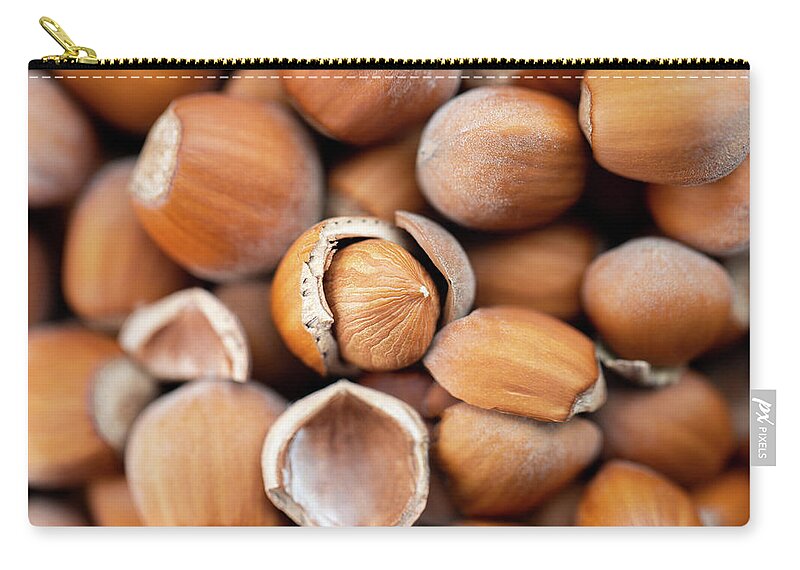The image displays a photo of numerous light brown chestnuts, focused on one prominently cracked chestnut revealing its pale brown nut inside. This photograph is printed on a small zipper-topped pouch with a gray label on the right side that says "PX Pixels." The chestnuts, mostly whole and oval-shaped, are scattered across the pouch in various orientations. Notably, alongside the cracked chestnut, there is a triangular piece of outer chestnut skin to the left and another curved opening from a different chestnut shell below it. The zipper atop the pouch is golden, and the stitching around it is clearly visible. The consistent light brown chestnut shells contrast with the paler, white-spotted recessed areas on the cracked chestnut, creating a simple yet detailed and textured composition.